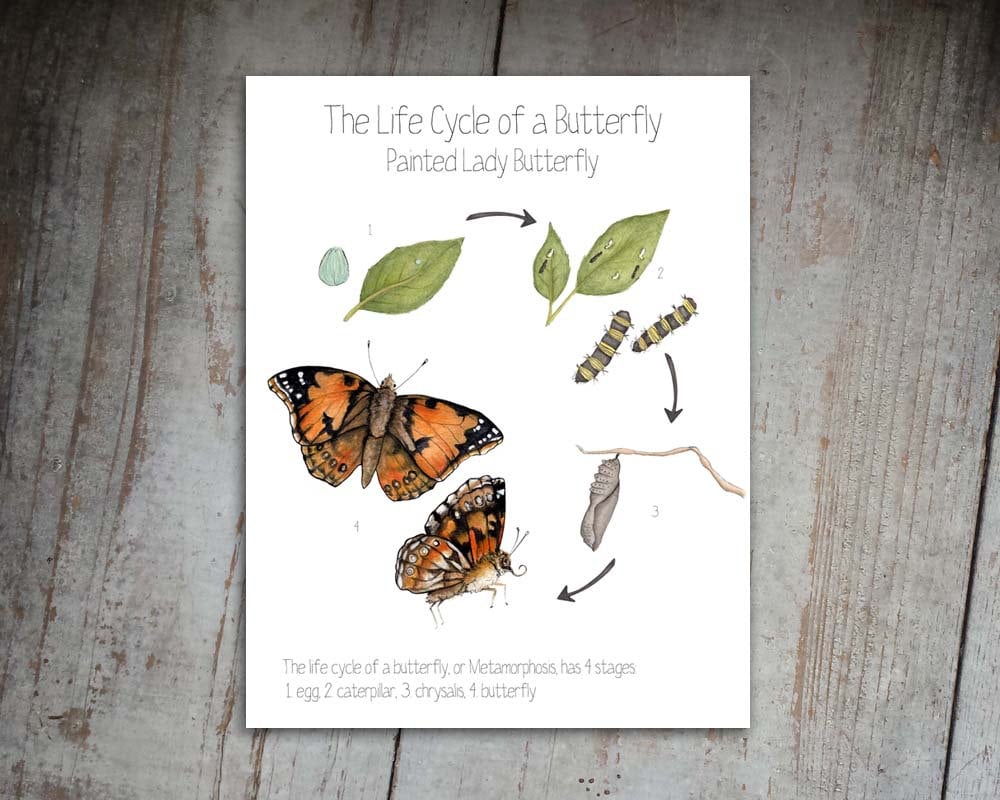The photograph features a detailed hand-drawn illustration on a white piece of paper, placed on an aged wooden table made of planks with light gray and brown stains. The paper is titled "The Life Cycle of a Butterfly. Painted Lady Butterfly" at the top in black text. At the bottom, it reads in gray, "The life cycle of a butterfly or metamorphosis has four stages: one egg, two caterpillar, three chrysalis, four butterfly."

The upper section of the paper displays a series of detailed depictions of each stage of the butterfly's metamorphosis arranged in a circular pattern with arrows guiding the viewer through the sequence. Starting in the upper left, a green leaf bears a small dot representing the egg. Moving right, the next stage shows white and black caterpillars on a pair of leaves. The illustration progresses to a close-up of a caterpillar, then down to a chrysalis hanging from a twig. Finally, the sequence ends with the butterfly, first seen from a side profile and then above with its wings spread open, shown from a top-down view.

Each stage is annotated with its respective number, matching the text at the bottom. Despite being hand-drawn in a slightly exaggerated style, the illustrations are fairly realistic and detailed, effectively depicting the life cycle of the painted lady butterfly.